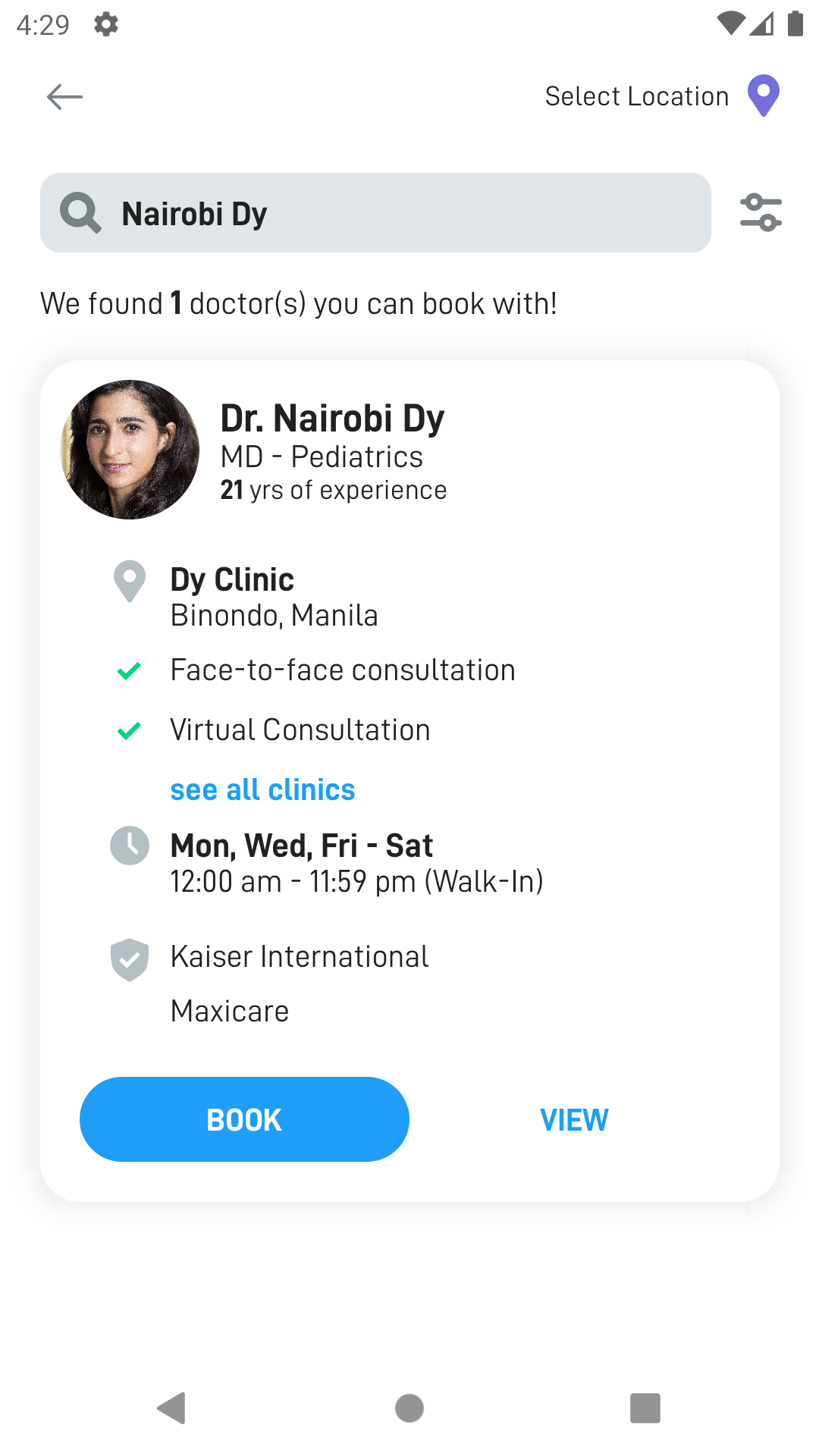The image depicts a mobile phone screen displaying a medical booking interface. In the upper left corner of the white background, the time is shown as 4:29, with a gear icon symbolizing settings to its right. On the far right side, Wi-Fi signal strength and battery level indicators are visible. 

Beneath this upper section is a dropdown menu labeled "Select Location," denoted by a blue pin icon. Following this menu, a gray search bar displays the text "Nairobi DY." The system has identified one doctor available for booking.

The doctor's information is presented in a gray-outlined rectangle. Within this rectangle, there is a circular image of a female doctor with black hair, accompanied by the text: "Dr. Nairobi DY, MD," noting her specialization in Pediatrics and her 21 years of experience. Below this is a gray pin drop icon indicating "DY Clinic by Natto Manila," followed by two green check marks indicating availability for both face-to-face and virtual consultations. An option to "See All Clinics" is highlighted in blue text.

Further details include a clock icon showing the doctor's working hours as Monday, Wednesday, and Friday through Saturday, from 12 a.m. to 11:59 p.m., with a notation indicating walk-in appointments are accepted. There is a verified check mark on a gray shield icon alongside the text "Kaiser International MaxCare."

In the bottom section of the displayed information, situated in the left corner, is a blue "Book Now" button, and to its right, the word "View" is highlighted in blue.